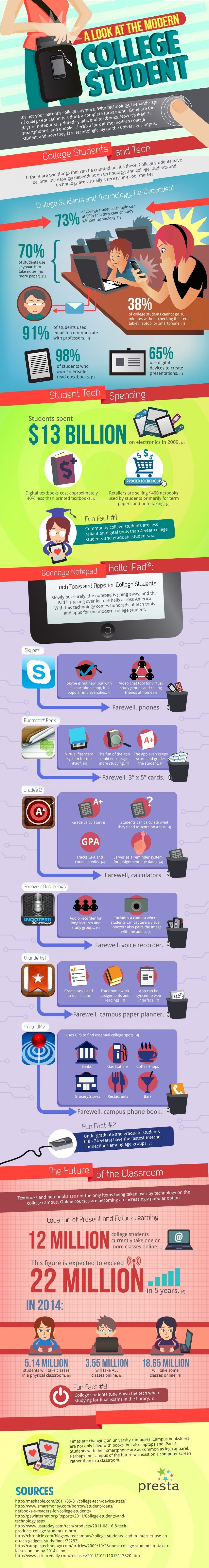The image is a digital infographic designed as a tall, narrow vertical banner that visually explores the technological habits of the modern college student. At the top, it features a light blue section with thin white lines and displays an illustration of a person dressed in a light orange shirt, blue pants, and a black cross-body bag, pulling out a tablet or notebook. This section is titled "A Look at the Modern College Student," followed by the subtitle "College Students and Tech" in a gray banner with white text.

Below this, there is a colorful display of statistics related to tech usage among college students, showing percentages like 73%, 70%, 91%, 88%, and 65%, though the accompanying text is too small to read. Moving further down, a large blue section highlights additional percentages (73%, 70%, 91%, 98%, 85%, and 38%) next to illustrations of a woman looking at her phone and a boy using a laptop. Following this, the infographic transitions to a bright green banner that states "13 billion" and provides additional unverifiable text details.

Next, a lavender section filled with various symbols and labels transitions into a reddish-pink area conveying significant data: "12 million" and "22 million in 2014," possibly referring to online course enrollment, though the exact context remains unclear. Near the bottom, further figures such as 5.1 million, 5.14 million, 3.55 million, and 18.65 million are presented. The bottom of the infographic lists sources and features the logo of the creator, a company named Presto.